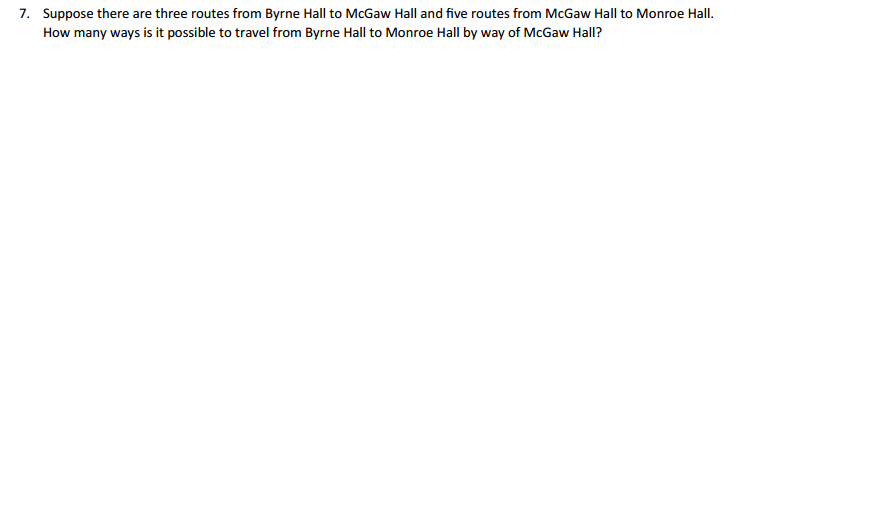The image captures a section of text displayed on a computer screen, against a stark white background. The text is numbered, beginning with "7." followed by a space. It reads: "Suppose there are three routes from Byrne Hall to McGaugh Hall and five routes from McGaugh Hall to Monroe Hall." 

On the following line, the text continues with a question: "How many ways is it possible to travel from Byrne Hall to Monroe Hall by way of McGaugh Hall?"

All instances of proper nouns are capitalized appropriately - "Byrne Hall" (with "B" in Byrne and "H" in Hall capitalized), "McGaugh Hall" (with "M", "G", and "H" in McGaugh capitalized), and "Monroe Hall" (with "M" in Monroe and "H" in Hall capitalized). The remainder of the page is blank, possibly intended as a space for writing an answer or simply highlighting the question. The text concludes cleanly, maintaining a focused, minimalistic composition.